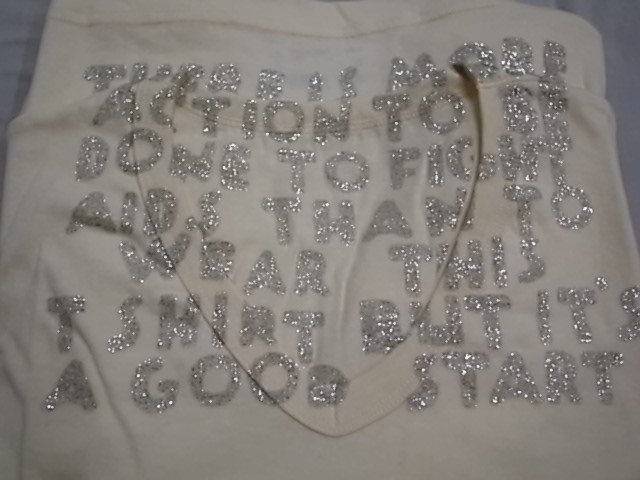Photographed against a neutral gray background, this image features a homemade white V-neck T-shirt designed for AIDS awareness. The unique design choice includes a message crafted with uneven, silver-glittered capital letters that are applied across the neckline rather than the front of the shirt. The lettering, though not uniformly glittered, conveys a powerful message: "THERE IS MORE ACTION TO BE DONE TO FIGHT AIDS THAN TO WEAR THIS T-SHIRT BUT IT'S A GOOD START." This handmade element adds a personal touch, emphasizing the importance of active participation in the fight against AIDS.